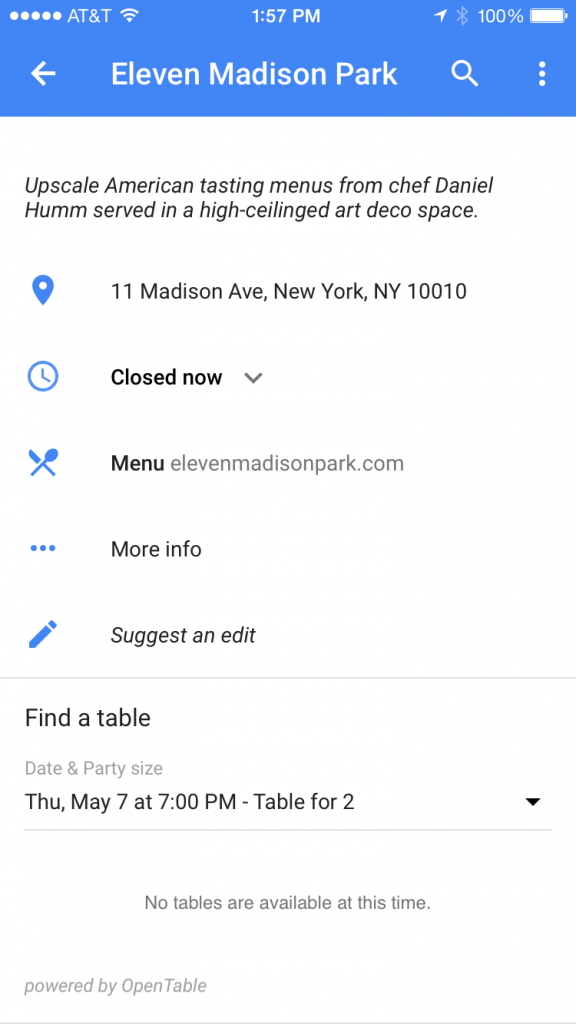**Descriptive Caption:**

A detailed screenshot of a mobile device displaying information about 11 Madison Park. At the top of the portrait-oriented image, there's a blue navigation bar with an arrow pointing left, indicating "Eleven Madison Park" spelled out, next to a magnifying glass icon and three vertical dots for additional options. Above this bar, the status indicators show the network provider AT&T, a full Wi-Fi signal, the current time (1:57 PM), an upward arrow, a faded icon, and a fully charged battery.

Below the blue navigation bar, there's a descriptive header with a white background that reads in italics, "Upscale American tasting menus from Chef Daniel Humm, served in a high ceiling art deco space." Under this header are five blue icons with corresponding text on the right:

1. An upside-down teardrop pin icon indicating the address: "11 Madison Ave, New York, NY 10010."
2. A clock icon stating "Closed now" with a downward-facing arrow for additional details.
3. A knife and spoon icon linking to the "Menu" at "elevenmadisonpark.com."
4. Three horizontal dots icon labeled "More info."
5. A pencil icon captioned "Suggest an edit" in italics.

A thin gray line separates this section from the reservation information below, which details "Find a table, date and party size" on "Thursday, May 7th at 7:00 PM - table for two." An empty center section notes, "No tables are available at this time." The footer of the image in the lower left corner, in italics, indicates "Powered by OpenTable," with a gray underline beneath.